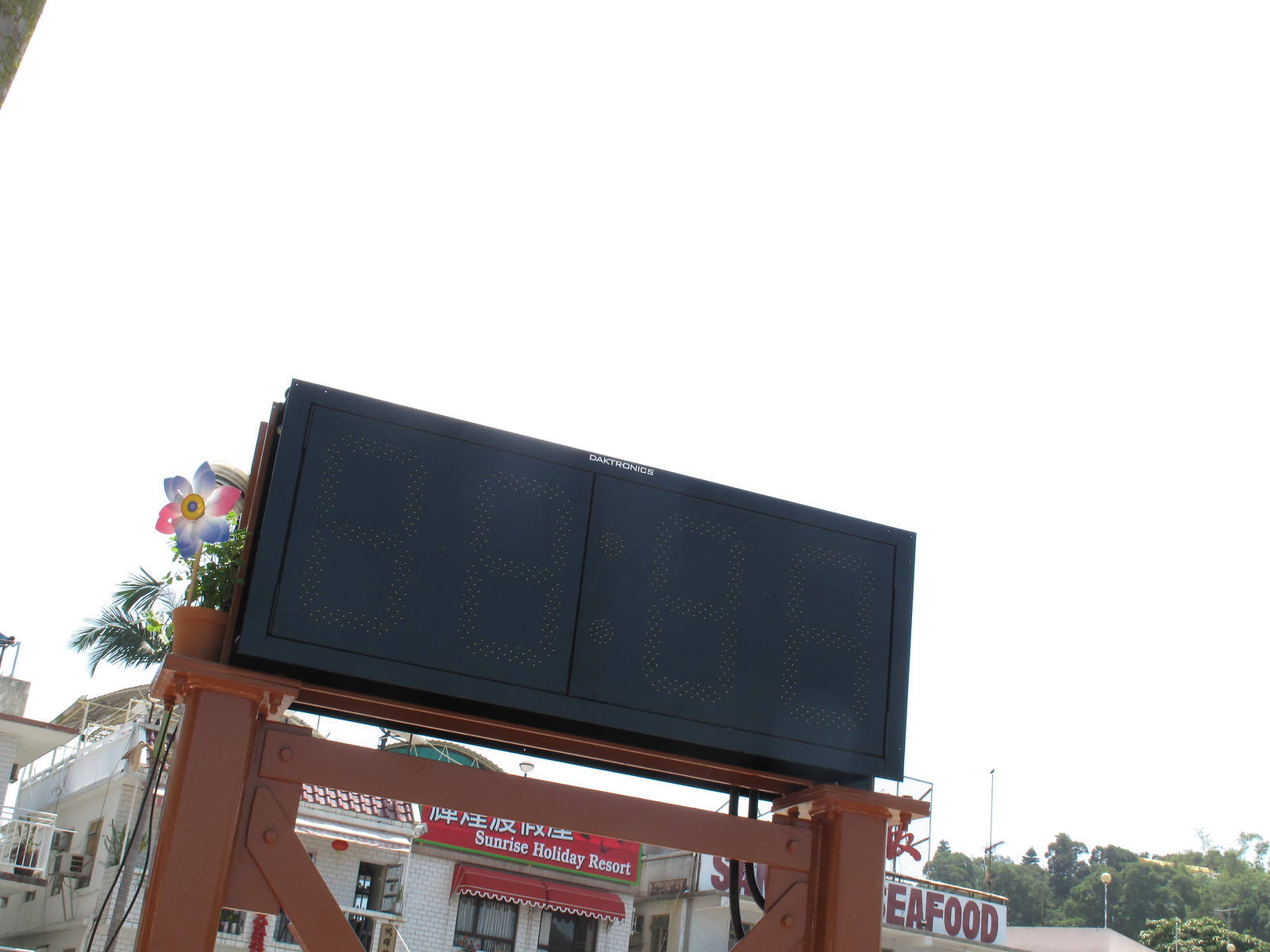This outdoor daytime photograph, taken with a slightly tilted camera, features a prominent rectangular digital display located just below the center of the image. The large black screen, which is currently off, has the faint outline of where numbers would display, indicating it is likely used to show time or temperature. The white text "D-A-T-T-R-O-N-I-C-S" can be seen at the top center of the screen. This display is mounted on a wooden structure with two vertical columns and a connecting horizontal beam, all painted brown. 

In the background, there is a one-story white brick building. The building prominently features Asian characters and, below them, the English text "Sunrise Holiday Resort," suggesting it may be a hotel. Additional signage indicates the presence of a seafood restaurant. The backdrop primarily consists of an overcast, white sky, taking up more than two-thirds of the background, with a green hill and trees visible in the lower right corner. Notably, there is a small blue and pink pinwheel flowerpot to the left of the screen. The photograph captures the front of the resort or restaurant with the digital sign as the focal point, set in a serene and sunny location.